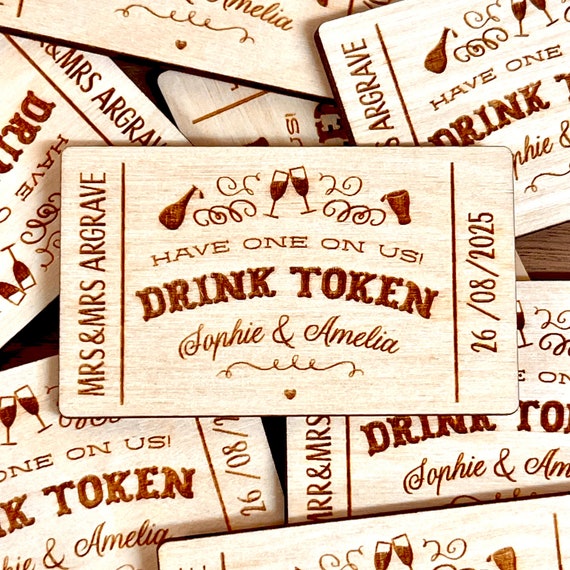This indoor photographic close-up captures a brown, rectangular wedding ticket card. Central to the image is an intricately detailed ticket with a blend of engravings and illustrations. On the left, a tilted wine bottle accompanied by whimsical squiggles sets a festive tone. At the heart of the card are two half-filled wine glasses clinking together in a celebratory toast, and to the right, a distinctively shaped upside-down triangular cup with a wide mouth and narrow base adds to the theme. 

The text is elegantly displayed across the card, starting with "Mr. and Mrs. Oggrave" arranged vertically. Horizontally centered, the card reads "Have One on Us!" followed by "Drink Token", with "Sophie & Amelia" beautifully underscored by a heart symbol. The date "26/08/2025" also runs vertically on the right side of the card.

Surrounding this central ticket are numerous identical cards, artfully arranged to give an impression of symmetry and artistic composition. Each card shares the same light beige wooden texture with deep brown engravings, ensuring the detailed elements visibly stand out. The overall scene evokes a meticulously planned celebration, ready to share joy and camaraderie among guests.